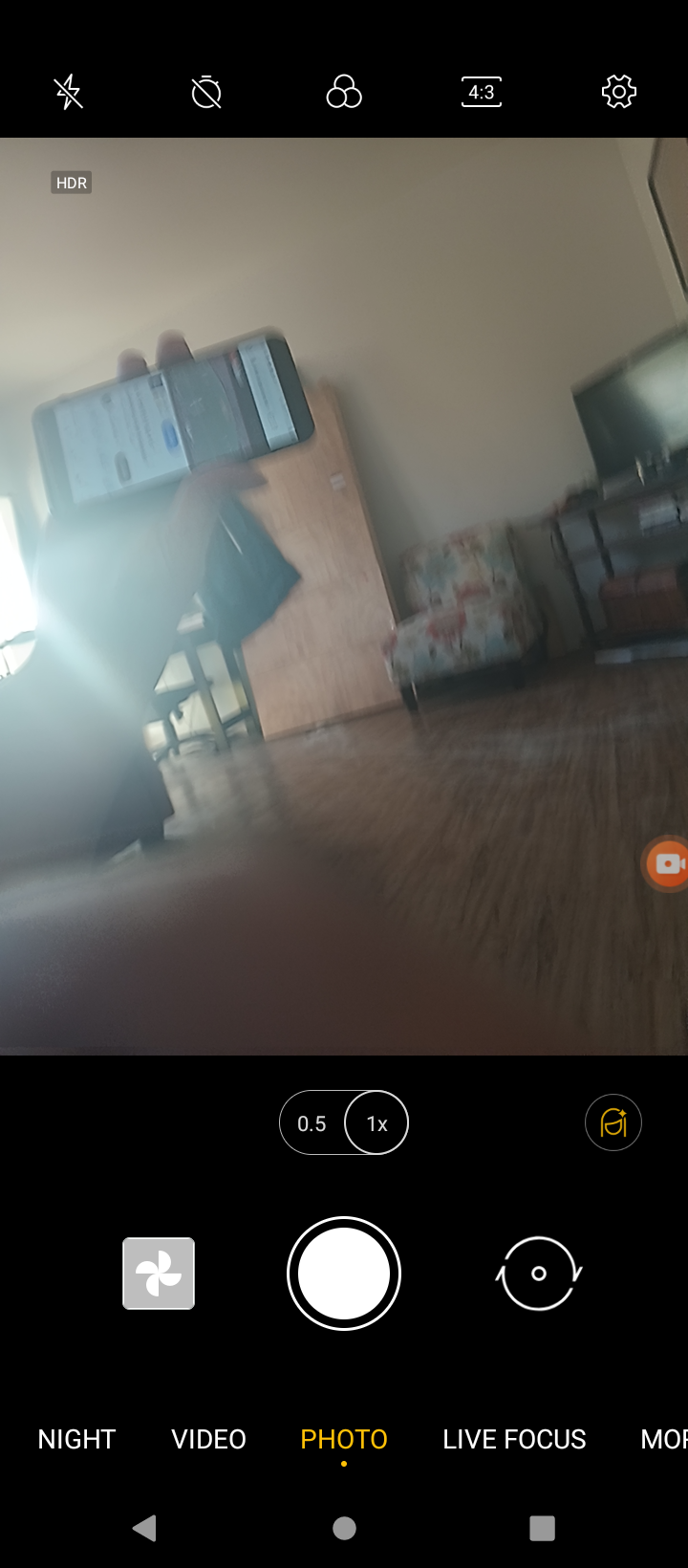This image is a screenshot from a phone's camera app, showcasing its interface while aimed at another phone that is in landscape mode. The phone being photographed has YouTube open, displaying a sports video with a green field and an advertisement. The screenshot captures the camera controls at the bottom, including options for night mode, video, photo, and live focus, with the central shutter button and a zoom slider ranging from 0.5 to 1x. The HDR option is indicated in the top left. The scene appears to be a standard living room with wooden or laminate flooring, a white wall, and a large brown cabinet. A black table is on the left, a floral print chair sits centrally, and a brown table with a TV or monitor is also visible. The living room environment is enhanced with details like an open door, adding depth to the setting.